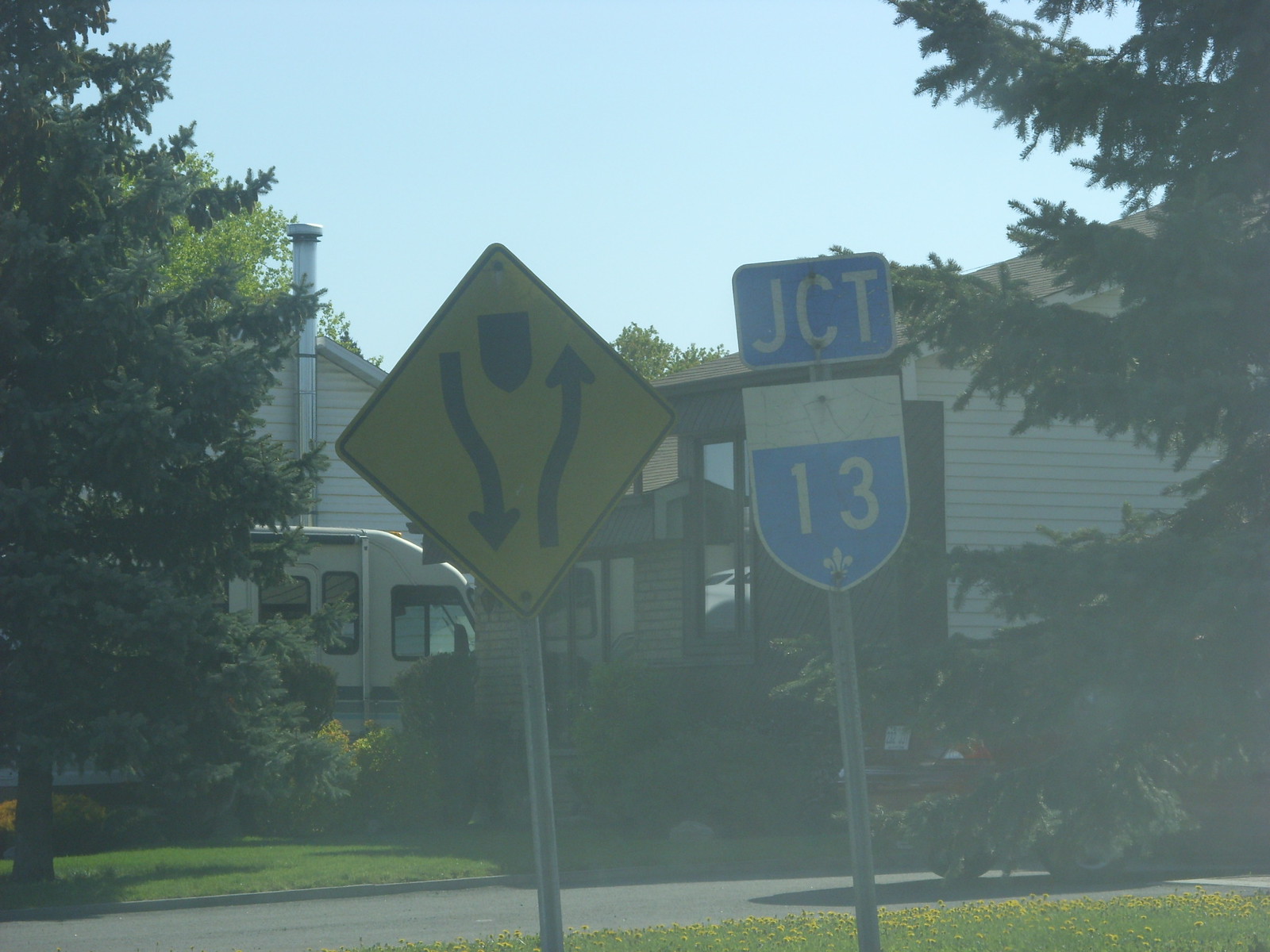In the foreground of the image, two prominent road signs stand tall. To the left is a yellow, diamond-shaped median sign, featuring a black arrow pointing down on the left with "median" in the center, and a black arrow pointing up on the right. Adjacent to it is a junction (JCT) sign, characterized by a blue and white color scheme. This sign has "JCT" at the top, followed by a shield shape colored white at the top and blue in the middle, displaying the number 13 in white, with a small fleur-de-lis at the bottom.

The background of the image reveals a residential scene. A red car and an RV are parked in a driveway, suggesting a well-kept suburban home. Green grass and an array of yellow flowers border the driveway, adding a splash of color. To the left, a large tree imposes its shadow over the front yard, while a similarly large evergreen tree stands on the right-hand side of the frame. Two houses are visible in the distance, with the blue sky overhead, free from any clouds, providing the perfect backdrop for this tranquil neighborhood scene.